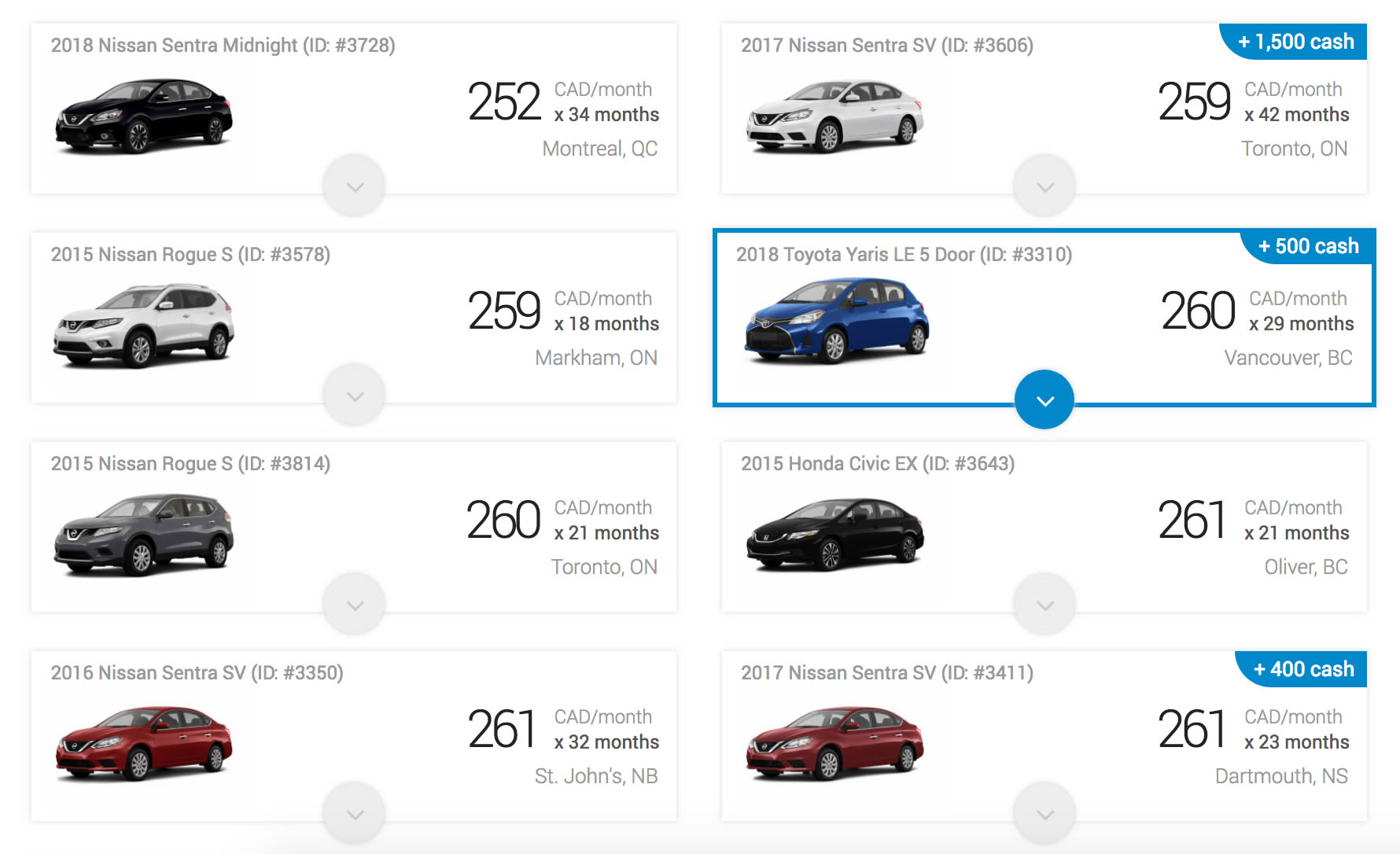A person is browsing on Cypher and evaluating a selection of vehicles for purchase. The screen displays eight cars, including a mix of sedans and crossovers, mostly from Nissan and Toyota. Specifically, the list features a 2018 Nissan Sentra (white), a 2017 Nissan Sentra, a 2015 Nissan Rogue (listed twice), an 18 Toyota Yaris LE 5-door, a 2015 Honda Civic, another 2017 Nissan Sentra (red), and a 2016 Nissan Sentra (red).

The user has highlighted the 2018 Toyota Yaris LE 5-door, which is priced at $260 CAD per month for a lease term of 29 months. The financial details for other cars vary slightly; for instance, the 2016 Sentra CV is listed at $261 CAD per month but for a term of 32 months, whereas the 2017 Sentra is available for a 42-month lease. Each vehicle is assigned a specific number, and the variations in months and payments are noted accordingly.